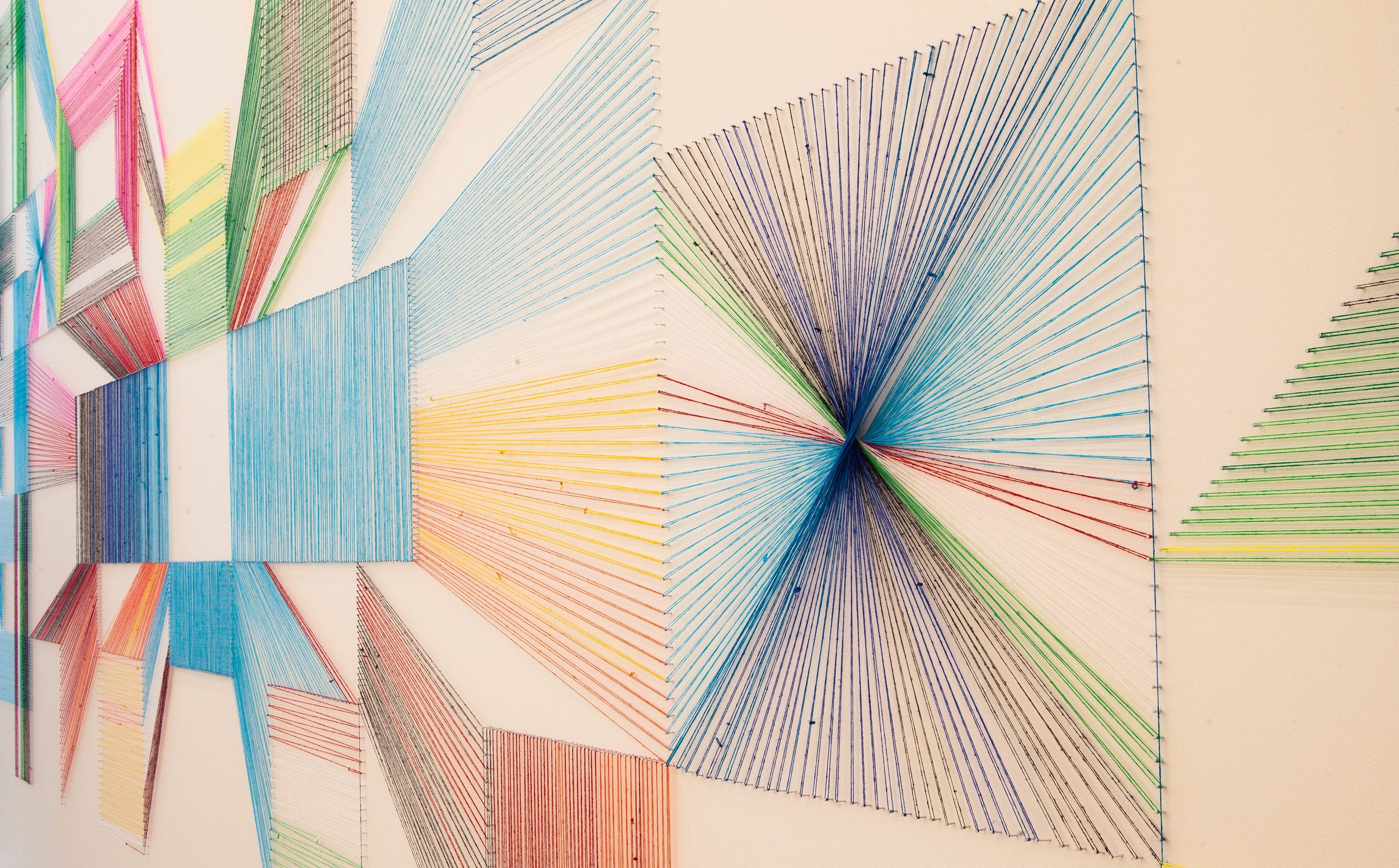In the image, we observe a detailed and vibrant art installation created with colorful threads stretched between nails placed on a wall. The right side of the image prominently features a large square where multicolored threads, including blue, purple, and red, radiate from the center to the edges. Adjacent to this square, at the extreme right, there is a half-triangle composed of green threads, with a notable yellow thread at the base, before tapering off with a final green thread.

The left side of the installation is densely packed with various shapes and patterns. There is a distinct pink artwork in the top left corner, amid an array of blue, pink, yellow, orange, and gray threads. These threads form intricate line designs that span the entire wall. As the lines spread towards the right of the image, they become more sparing until culminating in the large square of thread art.

The wall itself appears to be a neutral grey or peach color, which serves as a backdrop for this colorful display. The patterns on the left side of the image predominantly consist of rectangles and squares, with several small squares radiating out from a central rectangle. This visually striking piece effectively demonstrates a meticulous interplay of color and geometry, mounted onto the wall using nails or thumbtacks that hold the threads in place.